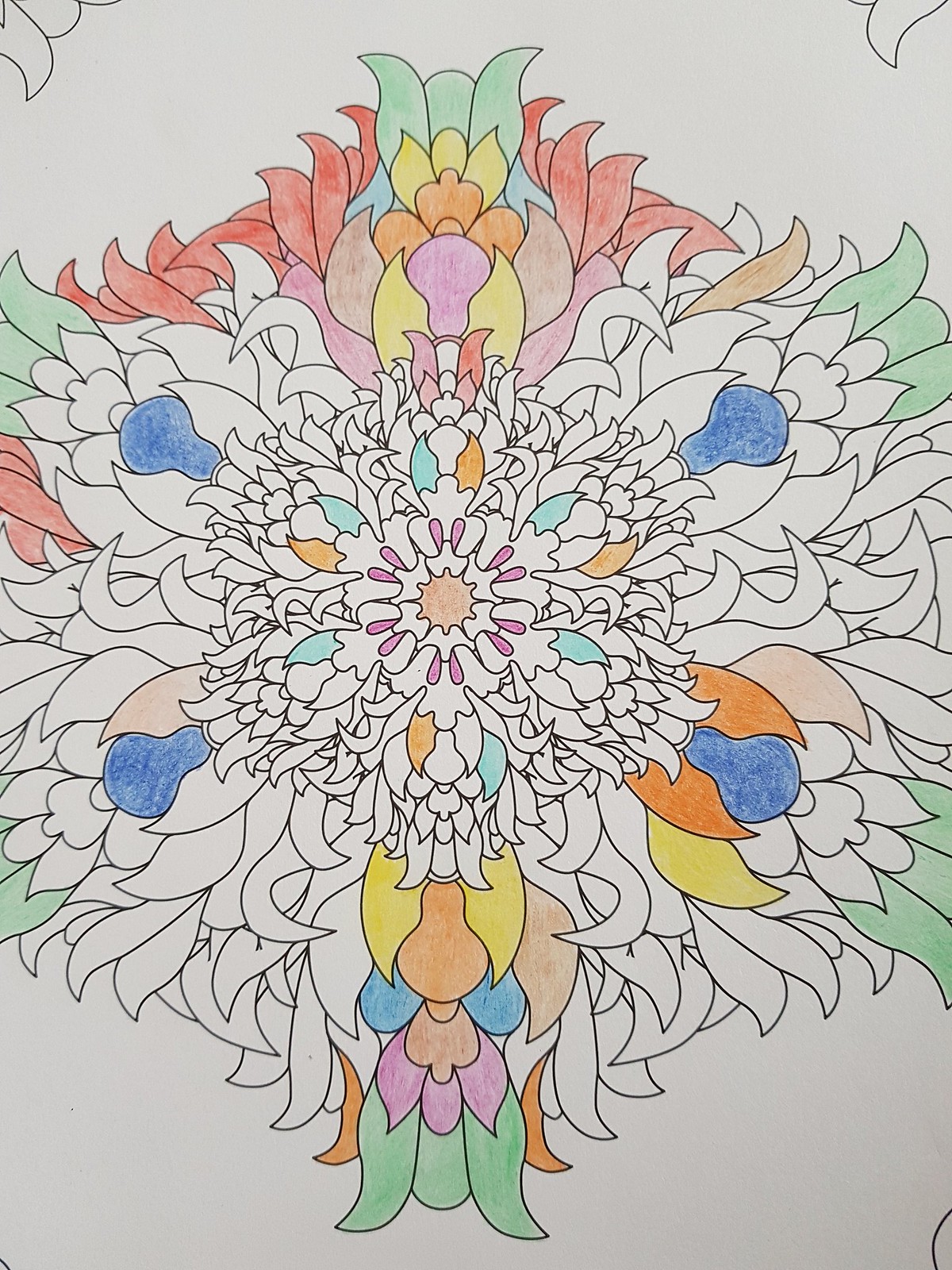The image is a partially colored, intricate drawing on light slate gray paper featuring an elaborate abstract design reminiscent of a flower or a kaleidoscope. It has a fine black outline, creating a detailed pattern with swirls and motifs that emanate from a central point. Some sections of the design have been colored in with colored pencils, showcasing a palette of rose, pink, orange, yellow, light green, royal blue, turquoise, and a darker blue. The coloring appears to be carefully measured, with petals and leaves grouped together in consistent hues. The artwork, about 15-20% complete, hints at a modern, imaginative interpretation that might even resemble stylized human figures within the abstract elements. It stands as an impressive work in progress, blending precision and creativity.